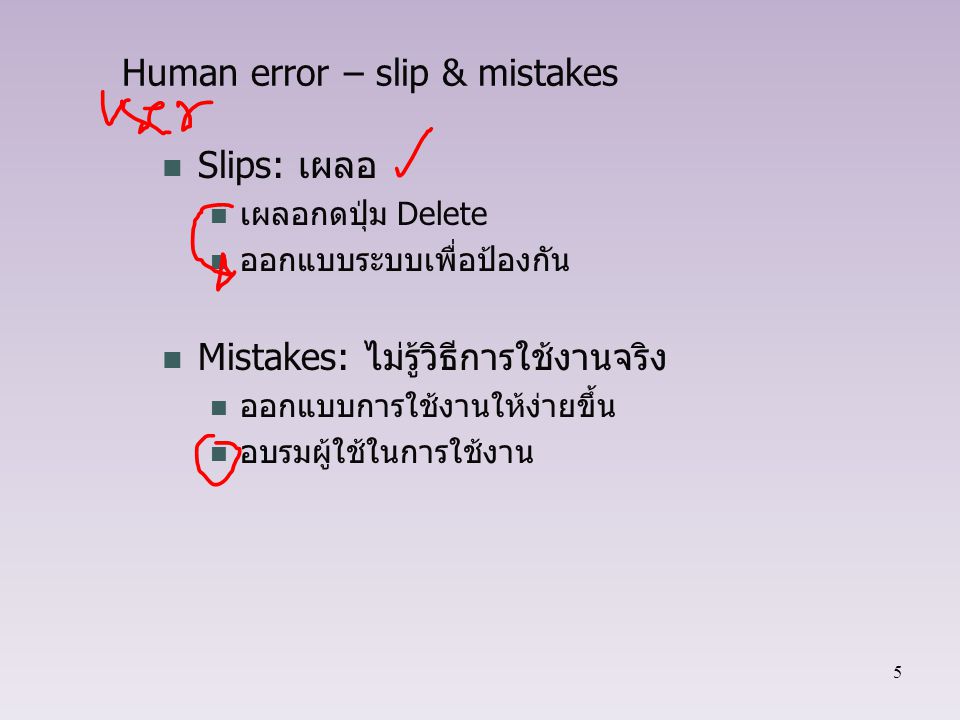The image appears to be a slide from an educational presentation, with a lavender gradient background that transitions from darker at the top to lighter at the bottom. At the top of the slide, in black text, it reads "Human Error - Slip & Mistakes," with the ampersand used instead of the word "and." Below this, there are two sections: one for "Slips" and another for "Mistakes." 

In the "Slips" section, a green bullet point marks the beginning, followed by foreign characters that are unrecognizable, except for the handwritten red words "user" and a check mark, all added over the original text. A red arrow curves from this section to the next.

Further down, part of the "Slips" section includes two more green bullet points with more foreign characters, one of which includes the recognizable English word "delete." Beneath this, the "Mistakes" section starts with a larger green bullet point, also followed by foreign characters, and continues with two additional green bullet points containing further foreign characters. Notably, the bottom green bullet point in the "Mistakes" section is circled in red.

The entire slide background is punctuated by a small black number "5" in the bottom right corner, suggesting that this is the fifth slide in a series.